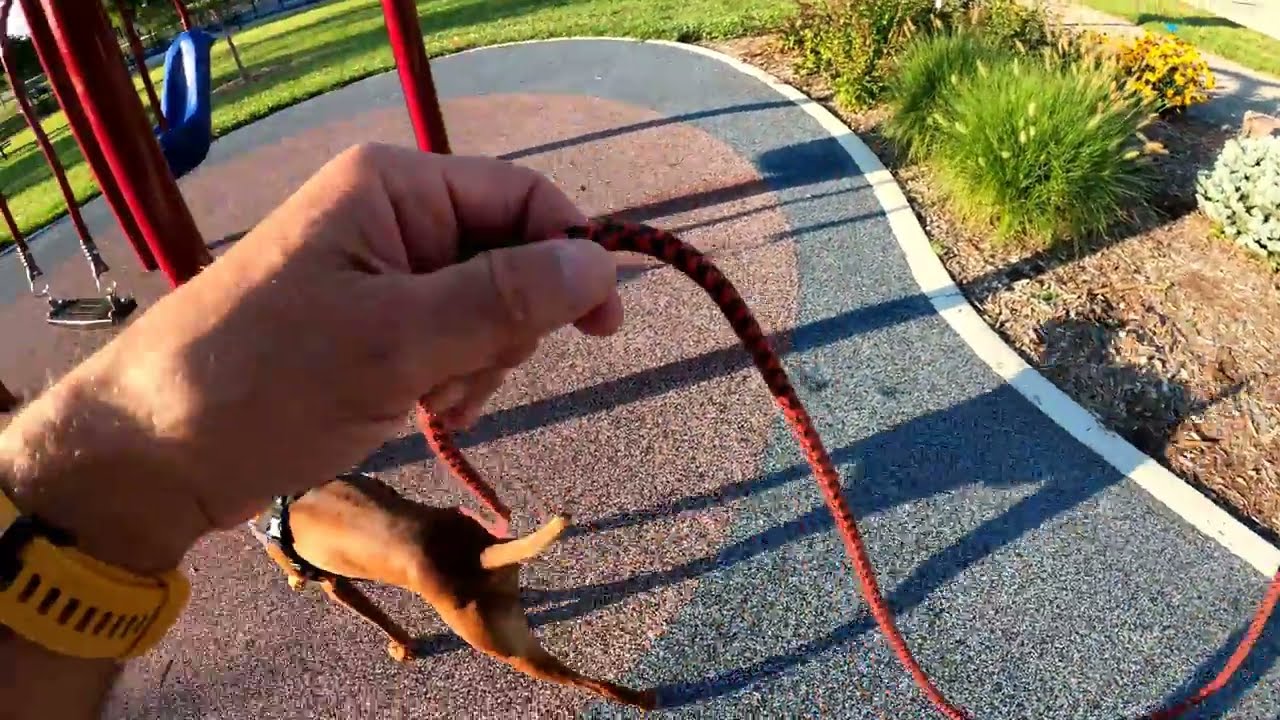In this image, a person is walking a reddish, skinny dog outfitted with a black harness and a green collar. The person, whose arms and hands are the only visible parts, is holding onto a red and brown checkered leash with both hands, adorned by a yellow watch band with a metal clasp. The pair is traversing a cracked, cement path bathed in bright sunlight, casting reflections off the pavement. Flanking the path are fields of green grass, interspersed with a couple of safety cones and a frisbee, with distant trees casting shadows. The scene vividly captures a sunny day, complete with crisp shadows and vibrant colors.